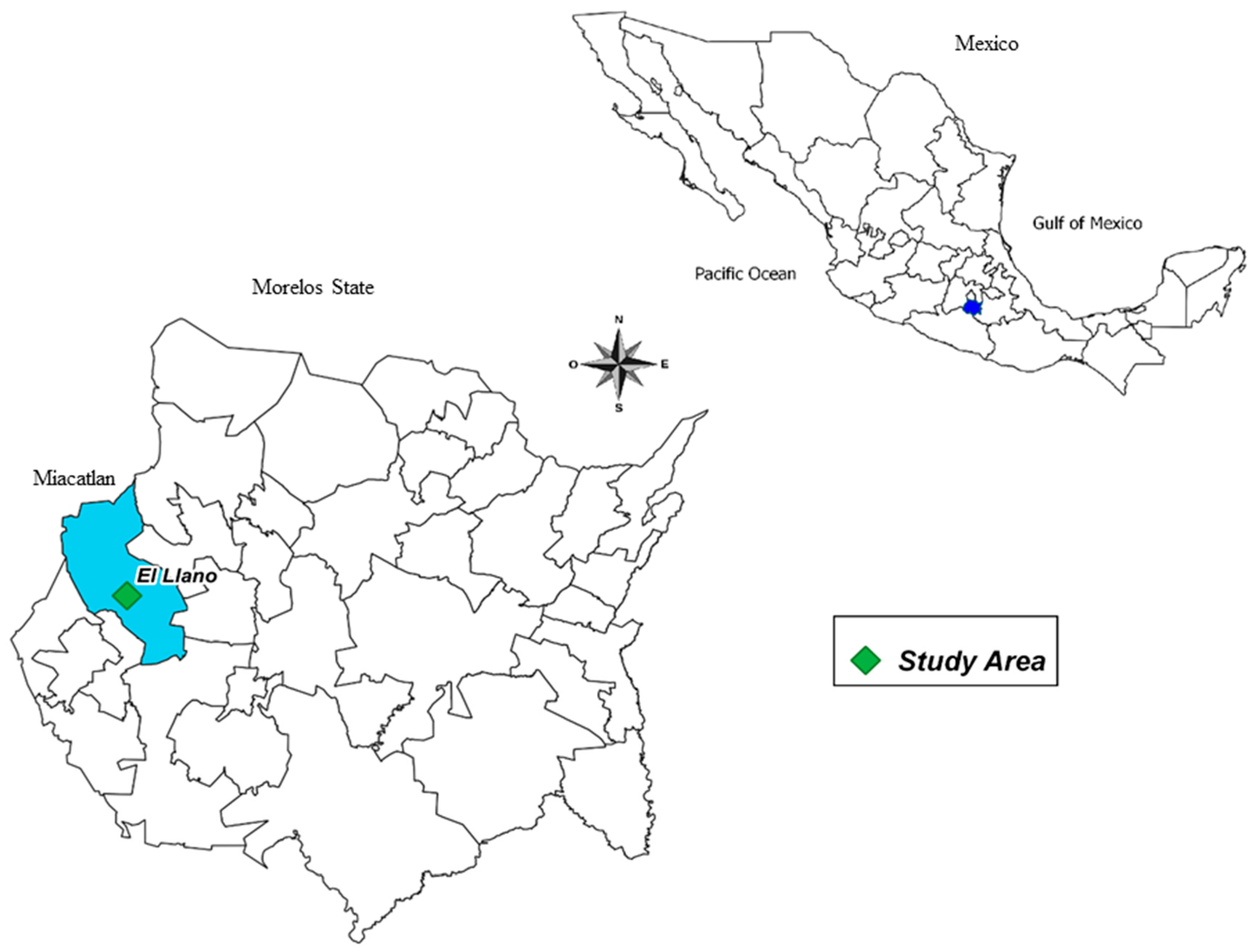The image is a detailed line drawing divided into two parts. At the top, there is an outline map of Mexico with all the states delineated. The Gulf of Mexico and the Pacific Ocean are labeled, and at the top, the country is marked as "Mexico." A blue dot appears in the southwestern part of Mexico, potentially indicating a specific point of interest. The central part of the image features a compass rose.

The bottom part of the image zooms into Morelos State, outlined in detail with boundaries likely representing municipalities. Among these, Miacatlán and El Llano are specifically labeled, with the area around them filled in turquoise. A green diamond (tilted like a square) within this region marks a study area, as indicated by a text box on the right. This text box suggests that the green diamond represents an ecological or scientific study area.

The overall layout has the Pacific Ocean named between the two maps, and the compass rose provides orientation. Despite the distinct marking of the blue dot on the Mexico map, its exact significance remains unclear due to the absence of a detailed legend. The more detailed map of Morelos includes informative elements such as bullet points and questions meant to guide the viewer's understanding of the study area.